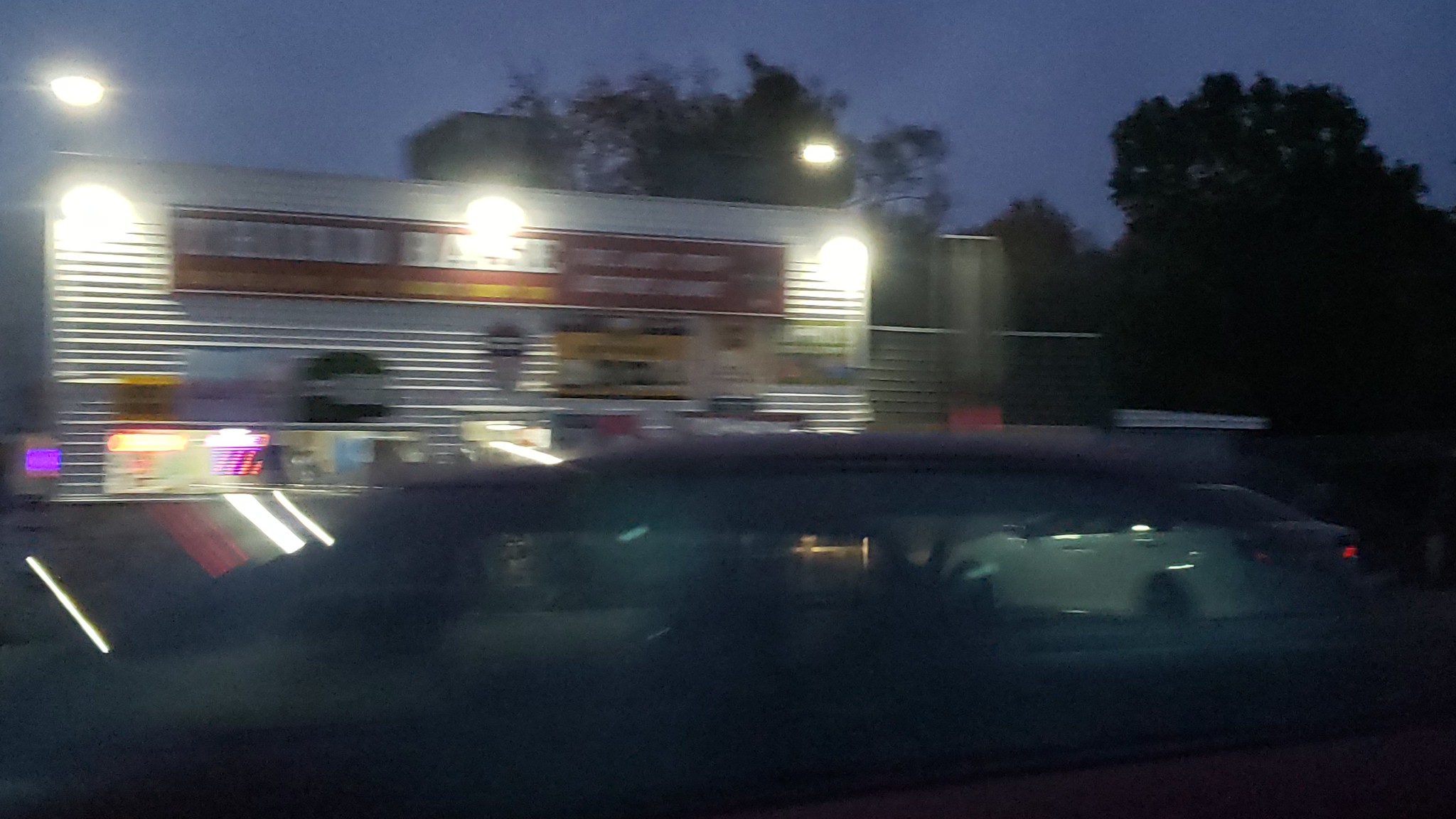This image, taken at night, features a blurred scene of a roadside diner or similar establishment. The photo is out-of-focus, making it hard to discern specific details clearly. Dominating the foreground is a large white car, parked facing the building in a parking lot. Another vehicle appears to be moving past the camera. The diner itself has metallic or clapboard exterior walls and is adorned with multiple signs, including a large red rectangular one with partially discernible white letters that likely spell "Bake." Additional signs in various colors and shapes, such as yellow rectangles with black borders and black signs with white letters, are present on the building. Three lights mounted along the roof illuminate the area. In the background, the indistinct outlines of tall trees are silhouetted against a very dark blue sky, indicating the photo was taken at dusk or night.